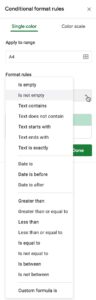The image depicts a significantly blurry and heavily cropped screenshot with a white background. Despite the blurriness, the text in the image is discernible, either in green or black. At the very top, the text "Conditional format rules" appears in black, accompanied by a black 'X' symbol to its right. Directly below, the phrases "Single color" and a partially legible "color something" can be seen. Beneath these, the word "Apply" is visible next to a dropdown box, identifiable by a calendar-like symbol to its right.

Further down, the section labeled "Format rules" includes another dropdown box, this time expanded to reveal its contents in detail. The expanded list within this dropdown exhibits a hierarchical structure, starting with seven items at the top, separated by a thin line from the subsequent group of three items. Another thin line delineates the next grouping of eight items, followed by a final single item at the bottom, each group distinctly separated by thin lines.